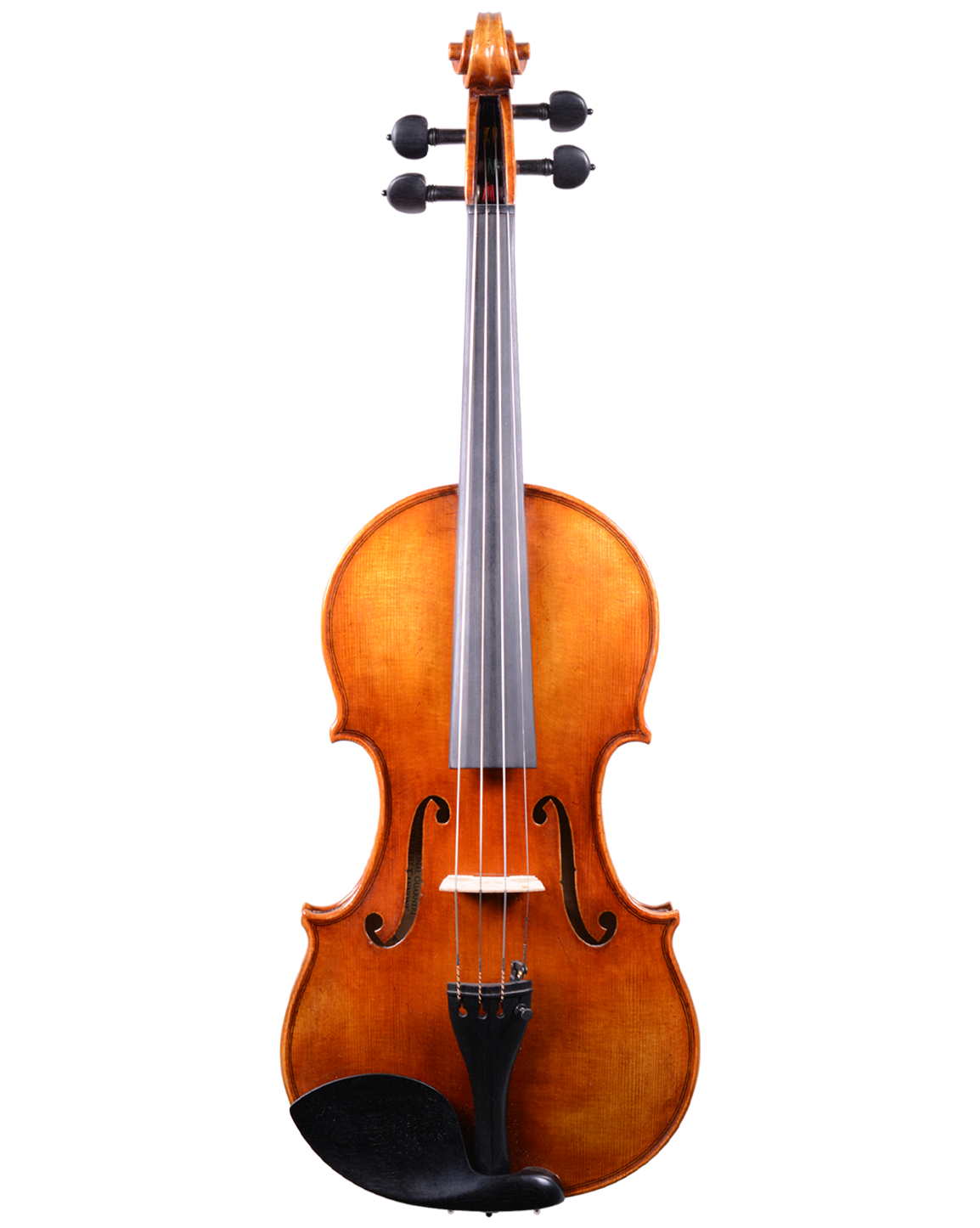The image depicts a clean and new light brown cello standing upright against a white background. The cello has a long handle or neck, with a gracefully curved wooden scroll at the top. The base of the instrument is shaped akin to the number 8, featuring two large curves connected by a thinner waist. The cello is equipped with four strings, anchored at the top by four black tuning pegs—two on each side of the neck. The area where the strings are played is darker, contrasting with the lighter wood of the body. Two elegant S-shaped sound holes are carved on either side of the strings, enhancing its intricate design. At the bottom of the cello, a black curvature component, likely the endpin, curves towards the body, adding to the sophistication of the instrument.